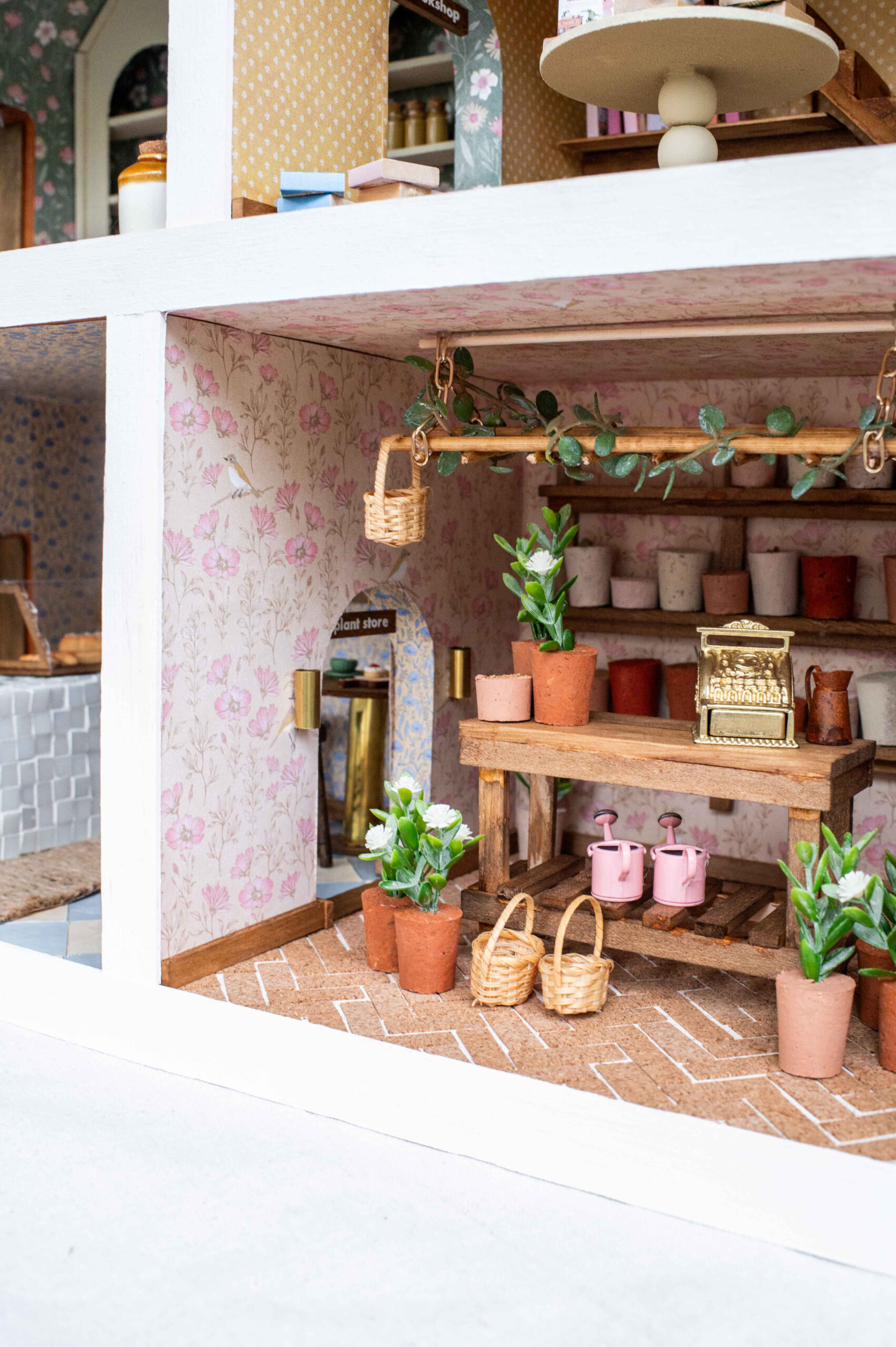This detailed photograph captures a miniature dollhouse segmented into different rooms, each teeming with intricate details. The central focus is on a larger compartment at the bottom right, representing a charming flower shop. This room is adorned with light pink, floral-patterned wallpaper and features an assortment of green plants in brick-like pots, with white flowers blooming from them. Two pots rest on the wooden floor, while two more are placed on a rectangular wooden table in the center of the room. The table also holds some golden rectangular objects, suggesting a commercial aspect. Beneath the table, a lower shelf supports two pink watering cans, adding to the gardening theme. The room's décor includes two woven wicker baskets on the ground and one hanging from the ceiling, enhancing its quaint, rustic vibe. Moreover, an old-fashioned gold till situated on the right side of the table emphasizes the room's commercial function as a plant store.

In the background, additional empty plant pots reside on shelves, hinting at a well-stocked shop ready for new arrivals. The dollhouse features three other rooms visible through open cubicles. The room to the immediate left seems to resemble a bakery, showing what appears to be baked goods inside a protective tray, possibly a loaf of bread. Above the bakery, another compartment displays what might be a collection of pottery items, though the details are indistinct. The room adjacent to the pottery area on the upper level resembles a study or library, furnished with a white table, bookshelves, and a set of stairs in the right corner.

This meticulously crafted miniature scene offers a delightful glimpse into a multifaceted dollhouse showcasing a flower shop, a bakery, and other intriguing rooms, each brimming with intricate details that evoke a sense of whimsical charm.